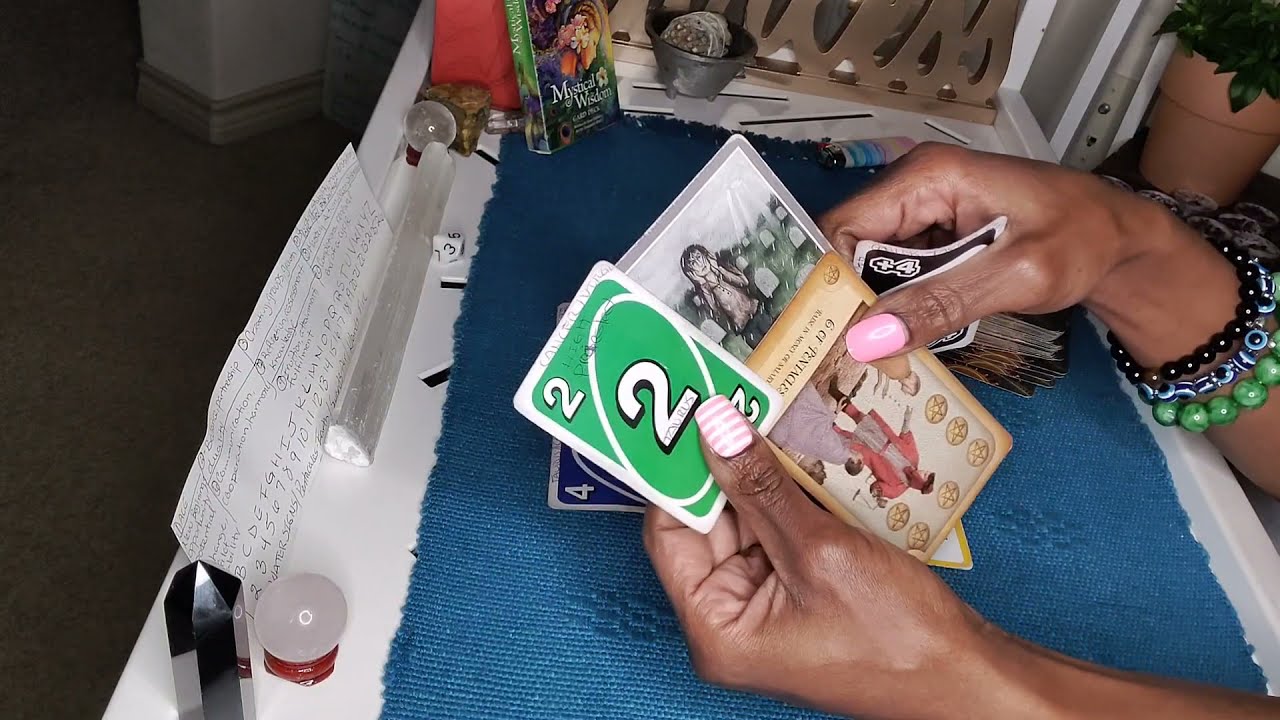The image depicts a woman with dark brown skin and painted pink fingernails, who is engaged in playing or manipulating various cards on a table. Her left thumb features white with pink stripes, while her right thumb is solid pink. She is adorned with beaded bracelets in black, blue, and green colors on her right wrist. The setting is an interior space under daylight, with a white wall, brown carpeting, and a flowering potted plant visible in the background.

The woman holds multiple cards, prominently displaying a green UNO card with the number 2 and an UNO "plus four" card. Among the assortment, there is a card illustrating a man with an anguished expression standing in what appears to be a graveyard. Another visible card has intricate details, showing a person in a red tunic surrounded by stars and interacting with others.

The table beneath her hands is covered with a blue mat. Surrounding her are various trinkets, including healing stones, a black crystal, a white sphere, and a twelve-sided white die. A piece of handwritten paper with alphabet and numbers, and a deck box marked "Mystical Wisdom," which suggests that some of the cards in use might belong to this mystical deck, are also seen. Additional objects like a rainbow-pattern cigarette lighter and other indistinguishable items add to the cluttered yet intriguing scene, evoking an air of both play and mysticism.